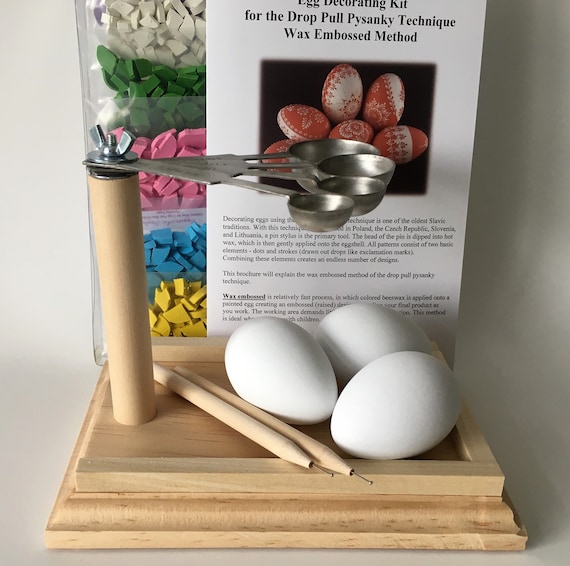This photograph features an egg coloring system set on a table against an infinity white background, giving the impression of the setup floating in white limbo. At the center is a wooden base, from which a cylinder extends upward, supporting four silver measuring spoons designed to hold eggs. On the base, there are three uncolored white eggs and two wooden pens with sharp metal tips. Behind these items, stacks of wax chunks in yellow, blue, pink, green, and white can be seen, stored in translucent plastic pouches. A piece of paper in the background provides context, reading "Egg Decorating Kit for the Drop Pull Pysanky Technique Wax Embossed Method," alongside a picture of brightly decorated eggs. The shadows cast by the items extend to the right, adding depth to the otherwise seamless background.